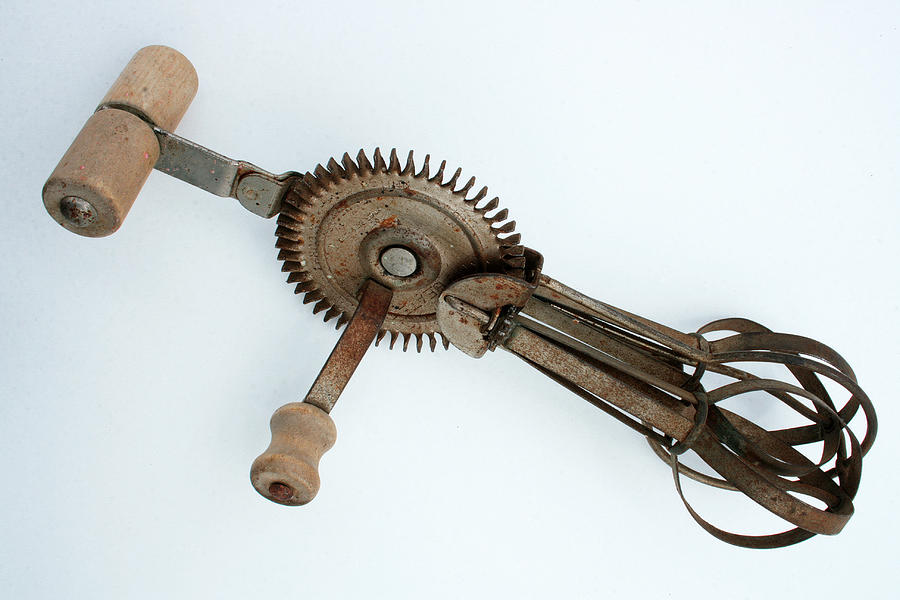This photograph, taken in landscape mode, showcases an antique hand-crank egg beater against a pale aqua backdrop. The vintage kitchen appliance features a wooden handle on one side, used to turn a large metal gear that engages with smaller gears to spin the steel beaters. A second wooden handle at the top allows the user to steady the device while cranking. The entire piece shows signs of heavy use, with significant rust covering the metal parts. This rusted finish adds to its antique character. Likely dating from the 1940s, this manual egg beater was an essential tool for mixing ingredients before the advent of electric mixers.